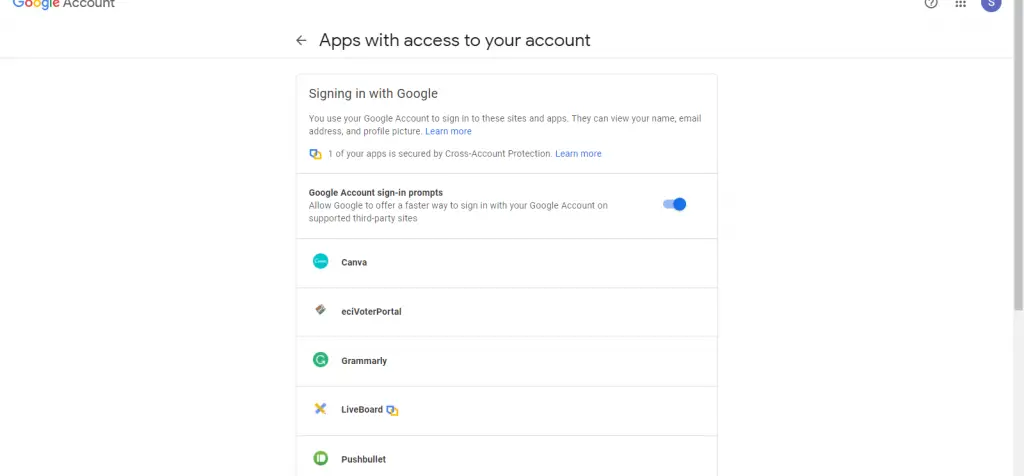The image depicts a Google account web page. On the left side, the Google logo and the words "Google Account" are prominently displayed. In the center of the page, there is a section titled "Apps with access to your account," though the list appears truncated. To the right, a partially visible menu adds an air of mystery by being cut off from the viewer's sight.

Below the main header, a boxed area labeled "Sign in with Google" is present. A disclaimer beneath this box instructs users on how to view their Google account by entering their name, email, and profile picture. Following this, the section offers an option to enable or disable Google account sign-in prompts via a toggle switch.

A detailed list of applications that have access to the account is presented beneath these instructions. The list includes several apps such as:

1. Canvas
2. Grammarly
3. Right Portal
4. Liveboard
5. PoshNet

Each of these entries signifies the permissions granted to various apps via the Google sign-in feature. The overall layout and the truncation of certain elements suggest a potentially comprehensive interface for managing app permissions and account security.